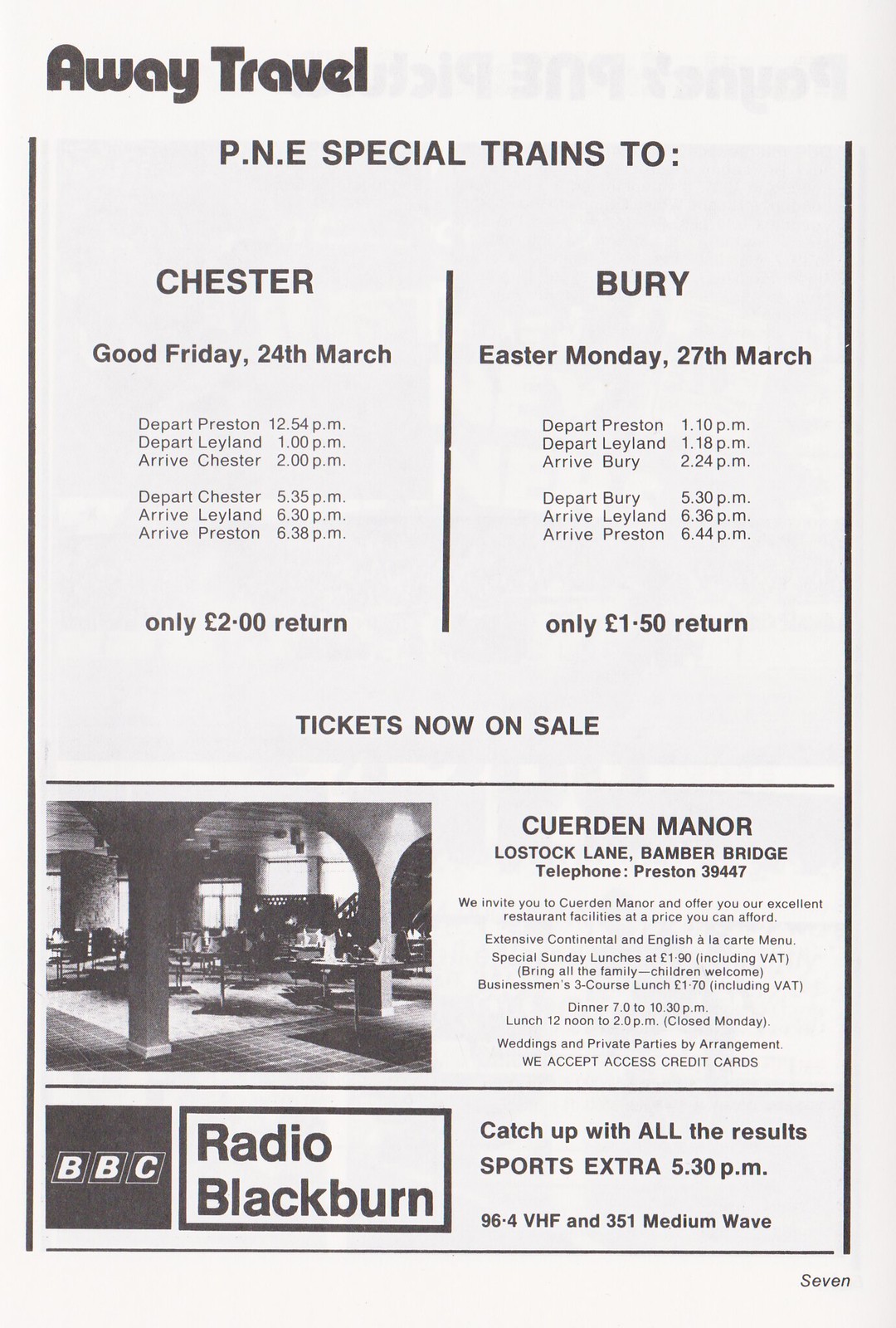This image, a scan from an old UK magazine or newspaper, prominently features a detailed schedule for "Away Travel" under the headline. The primary focus is on "PNE Special Trains" traveling to Chester and Bury. For Chester, the schedule lists departures on Good Friday, 24th March, from Preston and Leyland, with arrival and return times specified. The fare to Chester is £2.02 for a return trip. The Bury schedule lists similar details for Easter Monday, 27th March, with a return fare of 1.5 pence. Tickets for these special trains are marked as "now on sale."

Below this, a smaller ad for "Cured in Manor" at Low Stock Lane, Bramble Bridge, with a contact number of Preston 39447, indicates various services offered, though the low resolution makes specifics hard to discern. Next, a horizontally-aligned ad from BBC's Radio Blackburn announces "Catch Up with All the Results, Sports Extra" airing at 5:30 p.m. on 96.4 VHF and 351 medium wave. Lastly, the bottom corner of the image has the number "7" in tiny print.